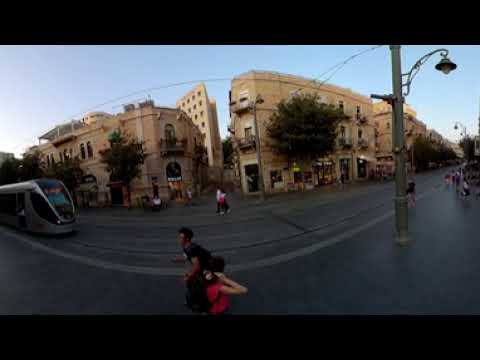The image portrays a city street scene captured with a fishbowl effect, creating a rounded appearance of both the sidewalk and street. Dominating the foreground, a dark-colored asphalt road curves prominently, accentuated by a white line that swoops from the left, dips down, and rises back up to the right. Centrally positioned are two individuals: a lady with lighter skin and black hair, wearing a short-sleeved red shirt, walking to the right with her arm bent near her ear; and a man with darker skin, black hair, and a black t-shirt walking in the opposite direction. 

A silver, futuristic-looking city bus with a sloped windshield is visible on the left side of the street, while on the right, a street lamp pole extends upward with wires protruding to the left and a hook bearing a light beneath it. The backdrop features multiple buildings, notably a light brown, three-story structure with a leafy green tree in front and a two-story building with arched windows. Additionally, a taller, lighter skyscraper with square windows rises behind them. The overall setting is outdoors on a bright day under a mostly blue sky with touches of white gleam near the buildings. The scene has no visible text and includes colors such as black, gray, red, tan, silver, pink, and green. The photograph includes borders at the top and bottom, framing the vibrant urban tableau.